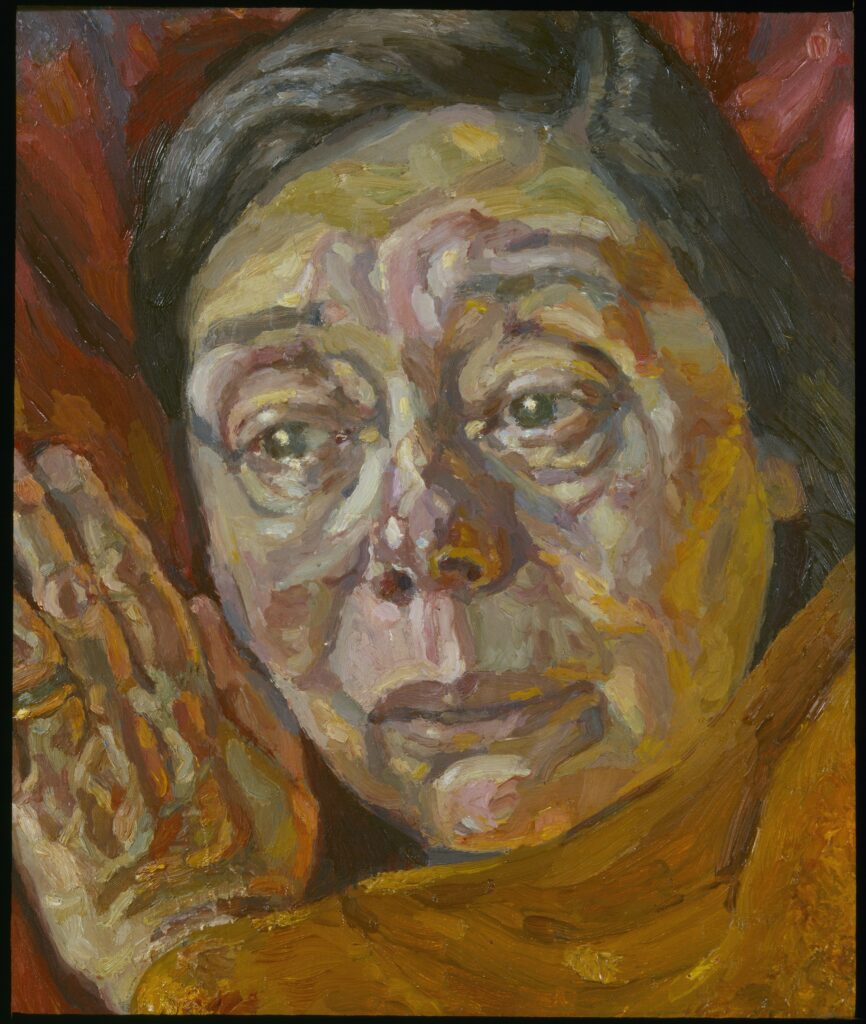This detailed painting captures the poignant image of a woman lying down with a deeply emotional expression on her face. Her dark brown, short hair frames her tanned and slightly flushed face, which holds a look of sadness as she gazes off into the distance. Her large, dark eyes appear somber, and there are hints of wrinkles, possibly intensified by her current sorrow. Her left hand, adorned with a golden ring, rests gently by her face, adding a tender touch to the scene.

The woman is surrounded by an orange-red fabric, which could be a pillow or blanket, adding warmth to the overall composition. This fabric extends to her upper body, contrasting with the yellow fabric that reaches up to her chin, possibly indicating a blanket she is wrapped in. The background and her skin tone show nuances of red and beige shades, suggesting the ambient light or reflecting her emotional state. The setting appears to be a bedroom or living space, lightly implied by the soft and intimate atmosphere, as she seems to be lost in thought, processing a moment of grief or deep contemplation. The artwork’s color palette of reds, neutrals, oranges, and browns further enhances the depth of her emotional state.